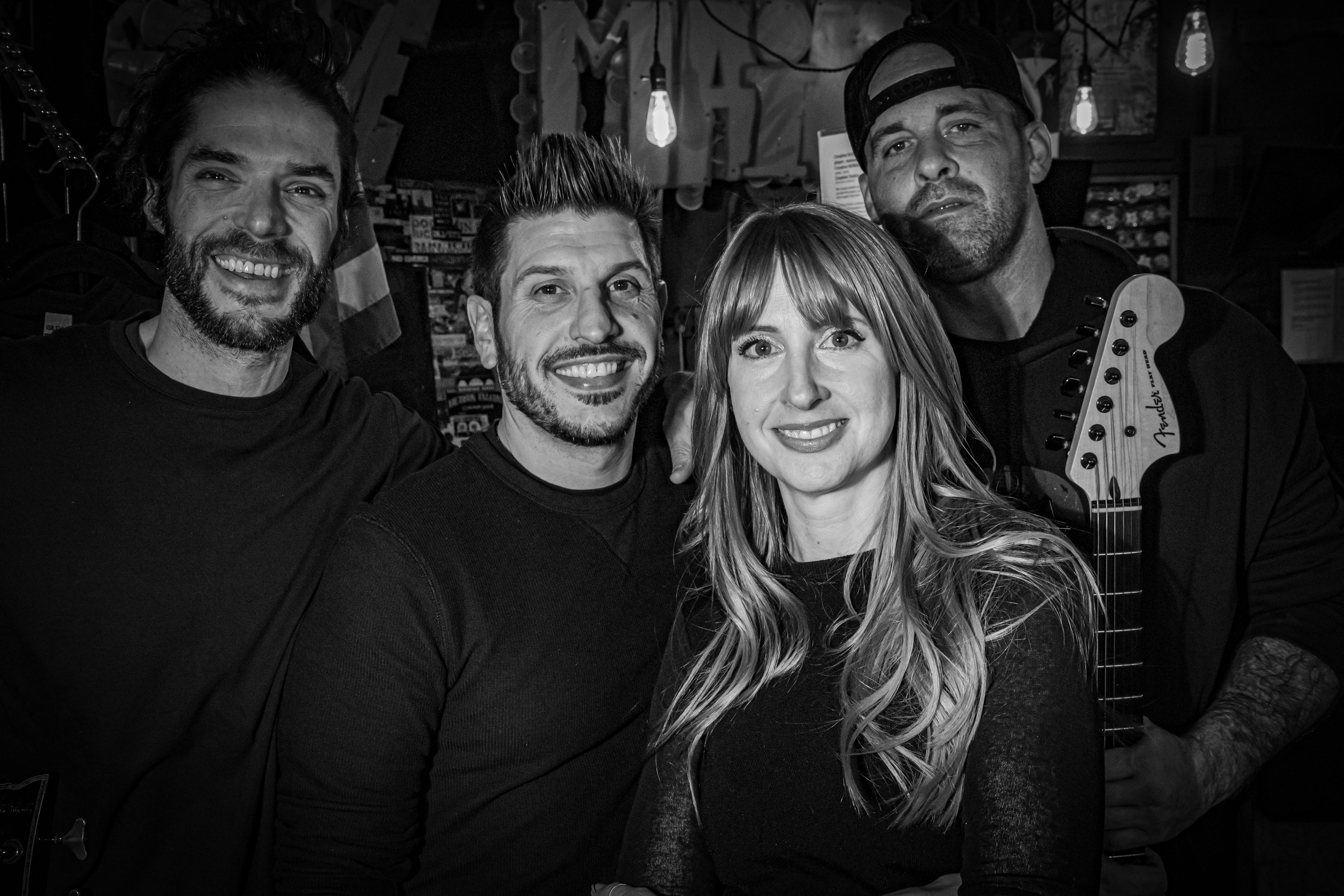In this black-and-white photograph, four members from the Rocket Shop Radio podcast episode of Big Heavy World stand side-by-side in a landscape orientation, all wearing black shirts. The man on the far left is smiling broadly, revealing his upper teeth, and has a black beard and mustache. Moving right, the next man also smiles widely, displaying a thin black mustache, a small patch of hair under his lips, and a spiked hairstyle. He has brown eyes and is mid-to-late 30s. Beside him, the woman in her 30s has long, flowing blonde hair cascading over her shoulders and down her chest, with a visible smile and brown eyes. On the far right, a man wearing a backwards black baseball cap and a thin stubble beard holds the neck of a Fender guitar; only the top part of the guitar is visible. He also has tattoos on his arms. In the background, a white light hangs from the ceiling on a black wire, along with other lights that are faintly illuminated, adding texture to the setting. The group appears to be looking up at the viewer, creating a lively and engaging promotional shot for the podcast.